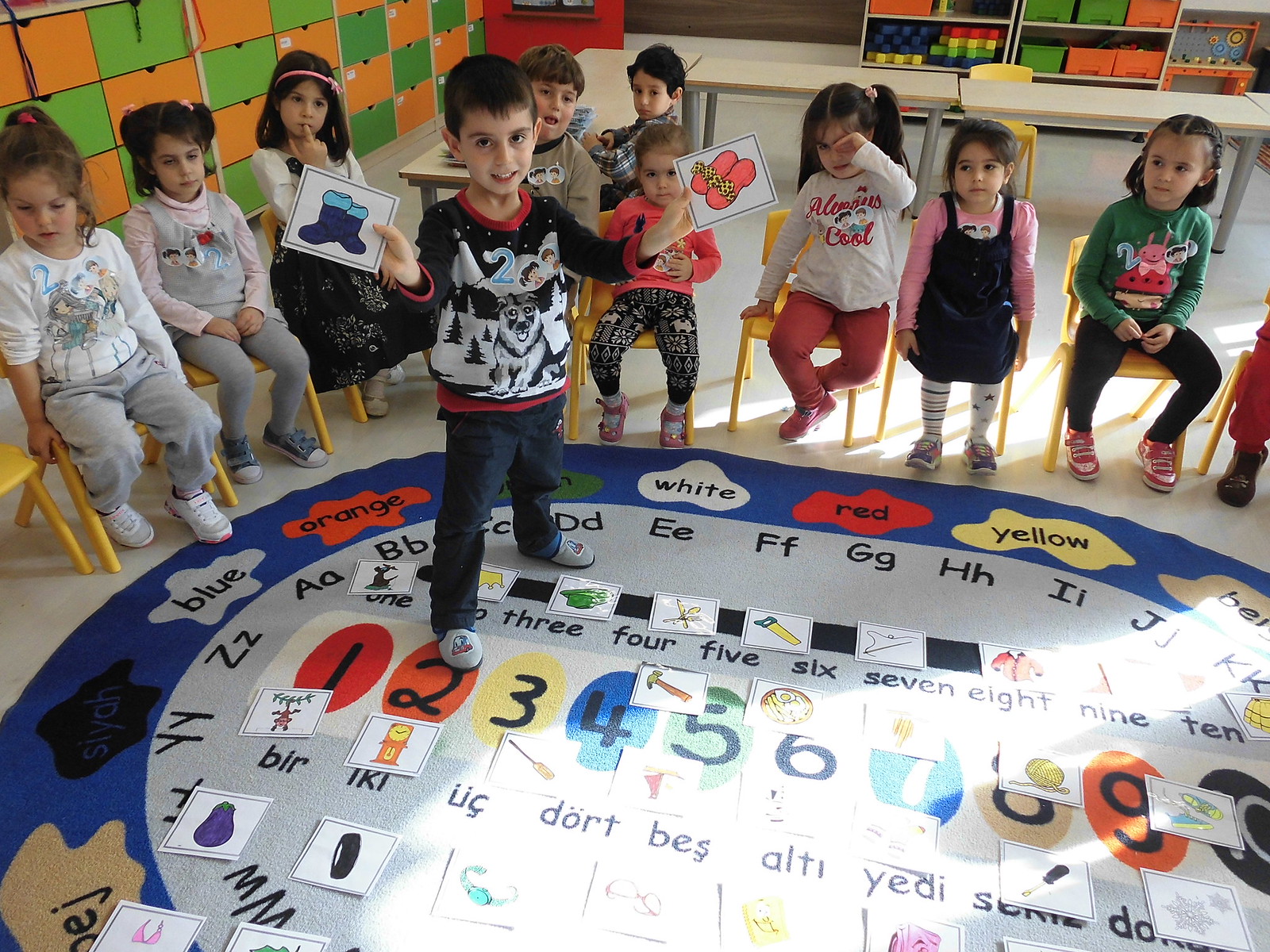This landscape-oriented color photograph captures a detailed scene inside a kindergarten classroom. Central to the image is a six-year-old boy standing confidently on a brightly colored rug adorned with letters and numbers. The rug features an array of colors, including blue, orange, green, white, red, and yellow, with an alphabetical border on a white background framed by a blue border decorated with red, yellow, and white conversational clouds.

The boy, looking up at the viewer, is wearing a distinctive black sweater with a red collar, embellished with a drawing of a dog and the number two. He pairs this with black pants and white sneakers. In his hands, he holds two colorful cards: one depicts purple boots, and the other shows pink sandals with leopard print straps.

Behind the boy, arranged in a semi-circle, are his classmates—six girls, seven girls, and three boys—seated in yellow folding chairs. The classroom is further detailed with a cubby wall on the left, showcasing bright green and gold cubbies in multiple rows. On the right, more school supplies are neatly organized with a table and chairs in front of them, adding to the educational setting. This photograph is a vivid representation of the classroom environment, reflecting a style of photographic representational realism that captures the nuances of kindergarten life.